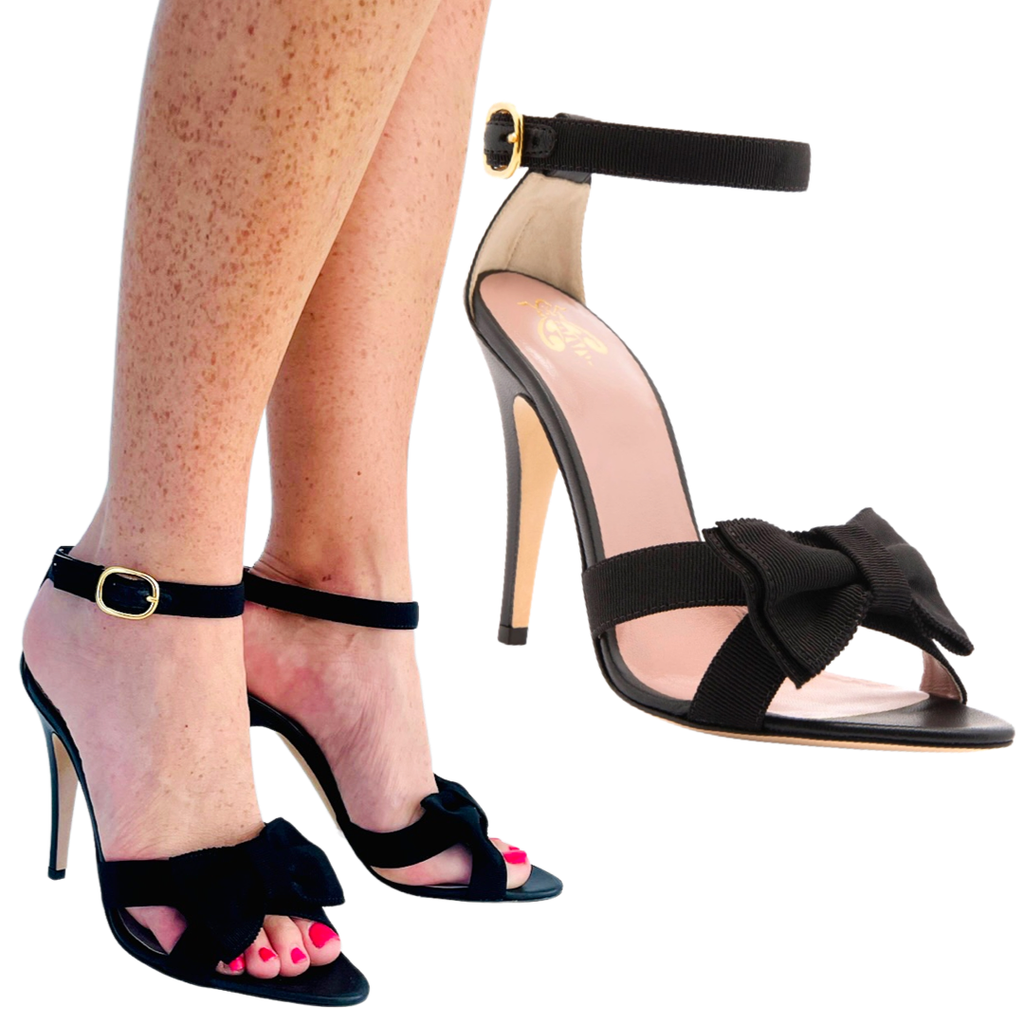The image depicts a Caucasian woman with freckled legs, emphasizing her pale skin. She is wearing high-heeled, open-toe black shoes that feature elegant design details. The shoes have ankle straps fastened with gold clasps and prominent black bows on the sections covering her toes. Her toenails are painted a vibrant red, adding a pop of color against the monochromatic footwear. On the right side of the image, there's a close-up of one shoe, revealing its brown inner lining, likely made of faux leather, and a bumblebee logo symbolizing the brand. The entire scene is set against a stark white background.